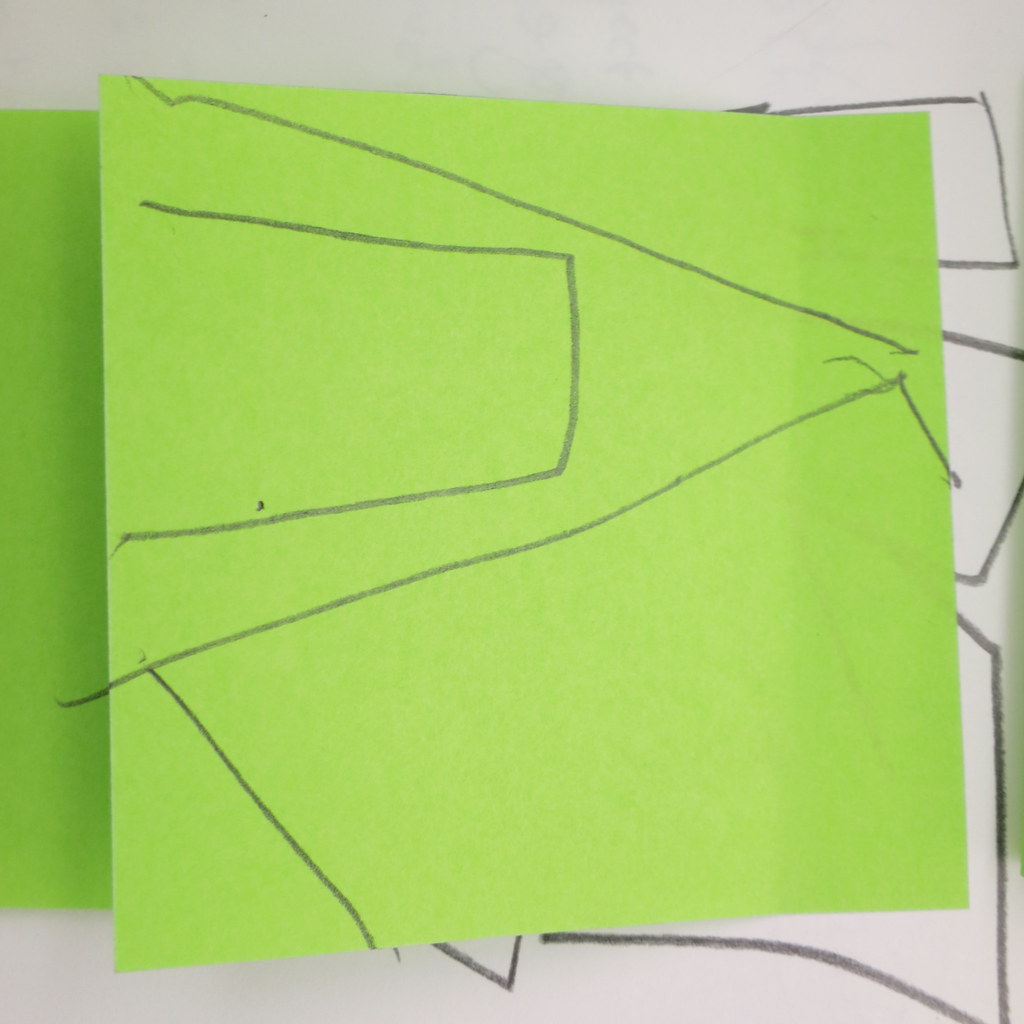In this vertical, rectangular photograph with a white or off-white background, there's a central focus on a sketch. At the center is a bright lime green square piece of paper, covering a portion of a smaller vertical rectangular green piece of paper beneath it, which is only visible along the left edge, about a quarter of the way down from the top and extending to a quarter of the way above the bottom. 

The visible part of the lower rectangular piece features a sketch with several intersecting lines: 
1. A diagonal line starts at the top left corner of the green paper and extends to a point slightly above the middle of the right edge.
2. Below it, a horizontal line begins about a third down the left edge, moves to the middle, turns vertically downward, and then extends left, ending slightly below the middle of the left edge.
3. Another diagonal line starts around three-quarters down from the top, slants toward the right side but stops short of the edge, and then continues in another diagonal closer to the right edge before reaching it.

Additional pencil marks are also found on the white background beneath the green paper:
1. One line starts from near the top right edge, goes horizontally toward the right edge, turns vertically down, then horizontally left, touching the green paper. This line seems to cast a shadow underneath the green paper.
2. Another line starts under the green paper, visible a third down from the top, runs rightward but is partially cut off by the green paper. It reappears midway down, making a slight diagonal toward the bottom right, ending about a quarter from the right edge, and then moves horizontally left, once again cut off by the green paper.
3. A final line starts about two-thirds down, moves slightly right, then vertically downward where it's interrupted at the bottom right corner, before continuing upward and reconnecting with the bottom middle of the green paper. A small V-shaped mark is visible nearby on the white background.